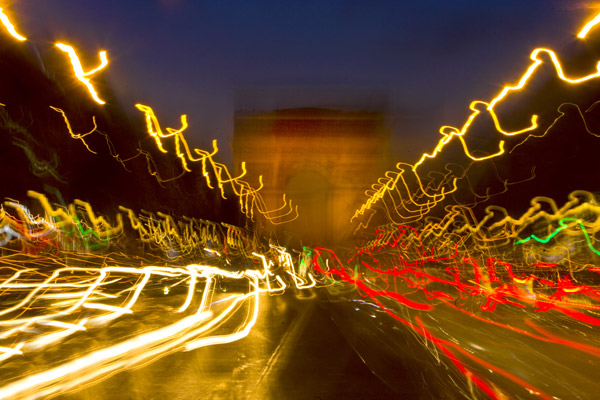A captivating time-lapse photograph taken at night showcases a large archway, reminiscent of the Arc de Triomphe, constructed from concrete. The sky in the background is a deep, dark blue, indicating the shot was captured after sunset. The image features a mesmerizing array of light trails created by moving traffic and possibly street lights, which stretch out in vibrant, repeated streaks of red, white, yellow, and hints of green. These light trails dominate the photograph, with white, yellow, and soft light orange as the predominant colors. The archway is set off in the distance, framed centrally by the camera's perspective. The lights, resembling irregular patterns of thin fluorescent bulbs, create an abstract overlay, adding an electrifying, almost surreal ambiance to the scene. The bottom of the image is punctuated with a gold, deep yellow tone, further enhancing the overall visual appeal.